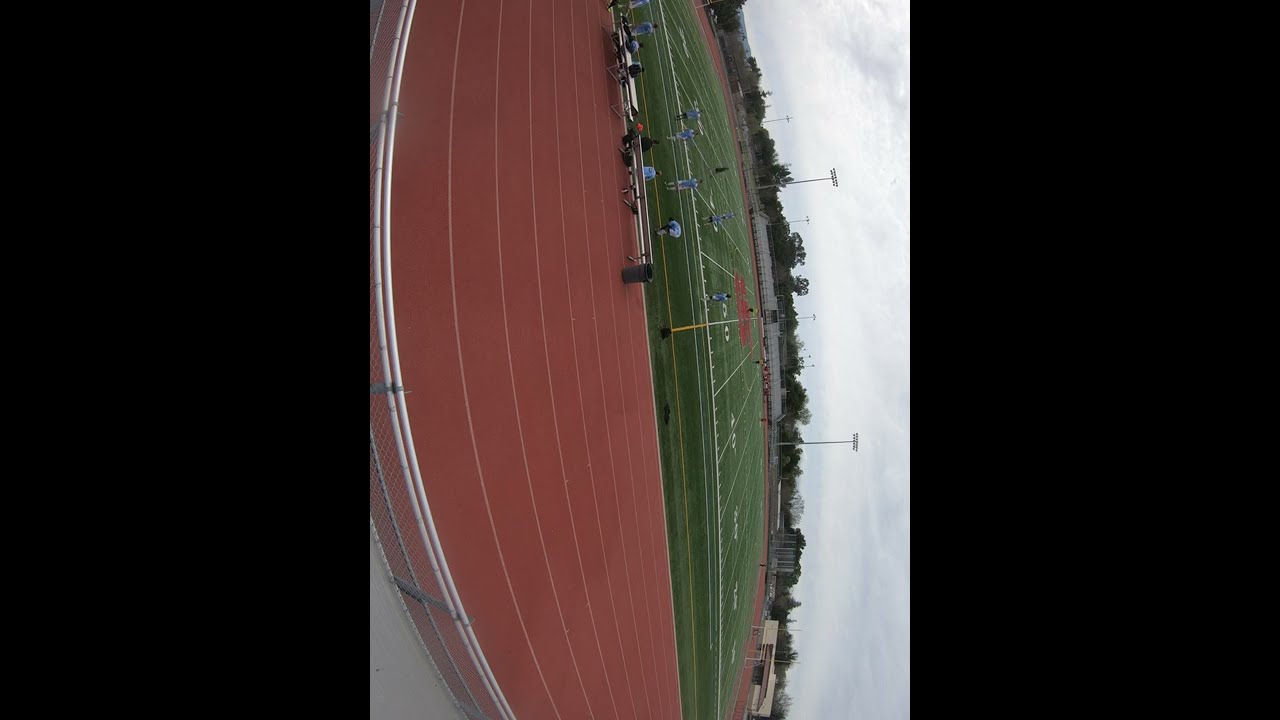The photograph is taken from behind the bleachers of an outdoor school stadium in daytime, with the orientation turned 90 degrees to the left. The image prominently displays a football field enclosed by an eight-lane red-orange running track. The field, with various lines and markings for football, has players in light blue jerseys scattered around, particularly near the 50-yard line. In the background, two tall stadium lights are visible against a cloudy sky. Surrounding the field are trees and a small building structure on the right. You can also see a chain-link fence around the track and a metal divider area, with a yellow pole and tiny flag or banner over it. Various objects are scattered on the field, though they are too distant to be identified clearly.